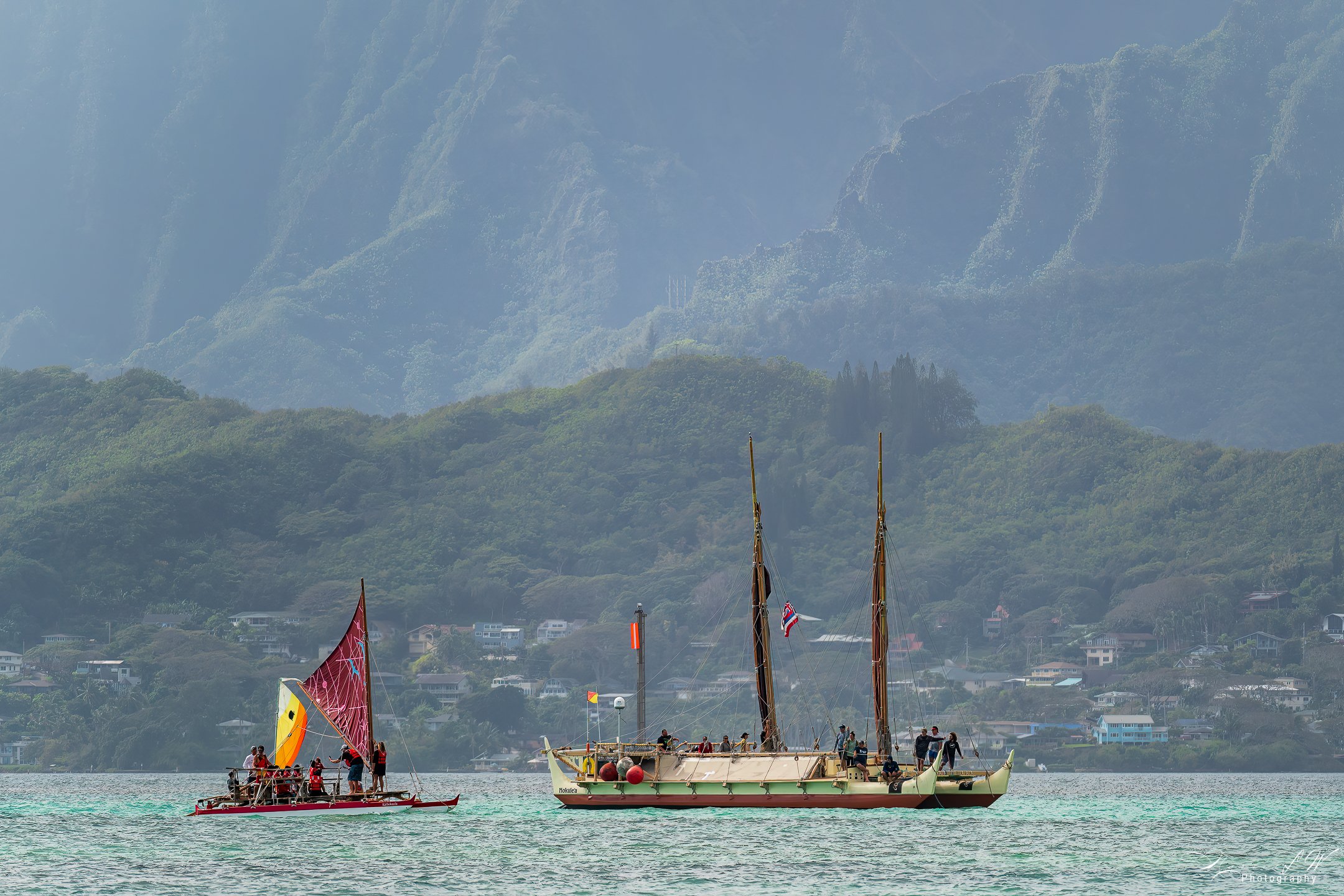The image features two sailboats navigating calm, light blue waters. The boat on the left is a smaller, red vessel, equipped with distinctive red sails and an additional smaller sail in orange and yellow, adorned with a black dot. This boat appears to carry approximately eight to ten passengers, positioned quite low near the water's surface. To its right, a larger sailboat roughly double the length of the smaller one, stands prominently. This bigger boat is a mix of very light green and white with touches of red on its exterior. It has folded sails and bears multiple masts along with orange and red flags, and a couple of red buoys. This vessel also hosts around ten individuals. 

In the serene backdrop, the scene is divided by a small green hill brimming with lush foliage and dotted with numerous buildings that likely constitute a nearby village. Looming behind this, a majestic mountain range ascends into the mist, their summits obscured by fog, presenting steep, sheer drops cloaked in dense greenery. The overall atmosphere suggests a nice sunny day with a hint of mist and fog, enhancing the picturesque quality of the landscape.